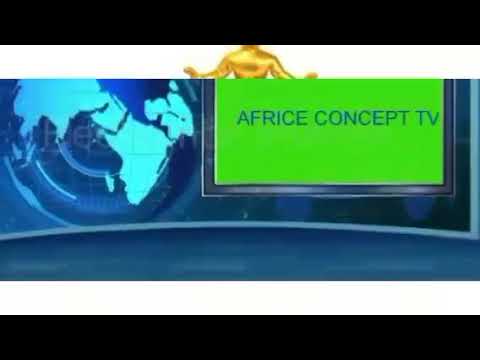This image is a wide, rectangular digital artwork or screenshot featuring several distinct elements that repeat across the descriptions. The top and bottom of the image are bordered by thick black bars, with thinner white bars adjacent to them. At the center, golden shoulders and outstretched arms—likely part of a statue—are visible, though the statue’s head is truncated by the top black bar. Beneath and between these white bars, a curved blue screen showcases an Earth graphic, predominantly in shades of blue, viewed from the Arctic Circle. To the right of this central blue section, there is a silver-outlined green rectangle with the dark green text "AFRICE CONCEPT TV." The overall style of the image is illustrative, and it appears to be a screen capture that perhaps serves as the opening screen for a media presentation or broadcasting outfit.